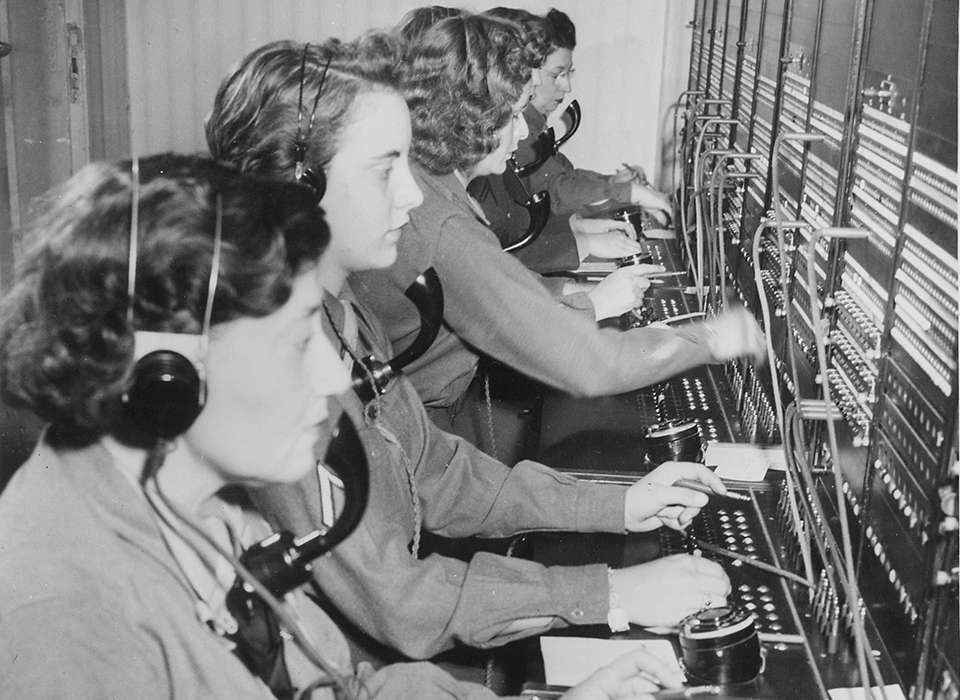This vintage black-and-white photograph, likely taken in the 1940s or 1950s, captures a row of four women hard at work at an old-fashioned telephone switchboard. The women are seated, facing to the right, and each of them is wearing a headset with horn-style microphones. Their hands are busy manipulating the circuit board in front of them, plugging in and rearranging cords to manage phone calls. Starting from the woman nearest to the camera: she has short dark hair and her finger is just visible near the switchboard. The second woman has short hair as well and holds a pencil in her left hand while working the board with the other. The third woman has short brown hair, wears a long-sleeve shirt, and is actively engaged with the switchboard. The fourth woman, positioned at the far end next to a white wall, has glasses and dark hair, also focused on the circuit board. In the background, there is a window with white blinds drawn closed. This scene evocatively illustrates the painstaking and detailed work of telephone operators during that era.